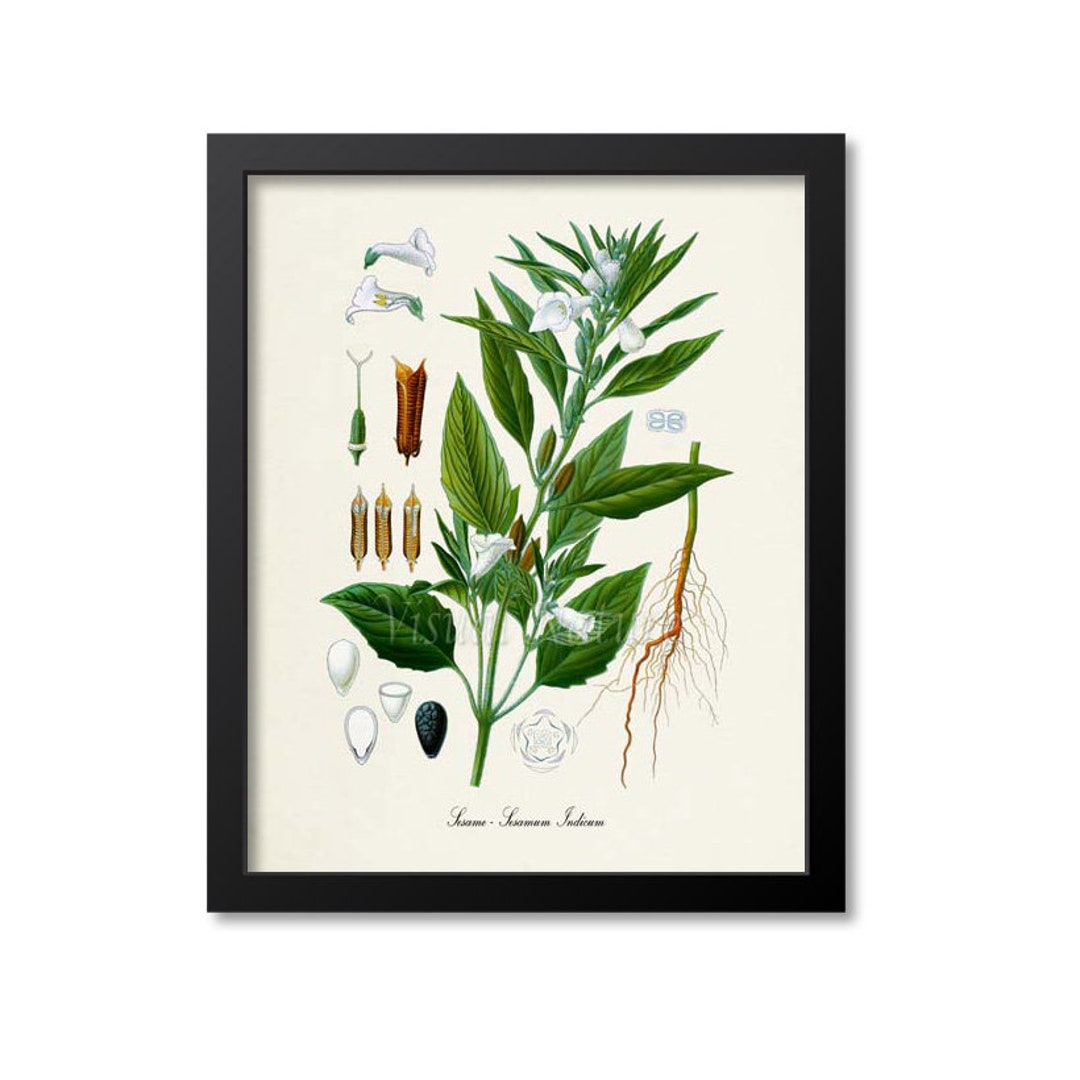A detailed, framed wall art in portrait orientation, showcasing a meticulously drawn daffodil plant, framed in dark walnut. The drawing, resembling a horticulturist's illustration, captures the entire daffodil plant, including its root system, stem, leaves, and white flowers in a stylized manner. The image is structured with different sections, highlighting various parts and angles of the plant on the left side, while the right side displays the comprehensive root system. The off-white paper background is bordered in black, emphasizing the intricacy of the detailed botanical study.